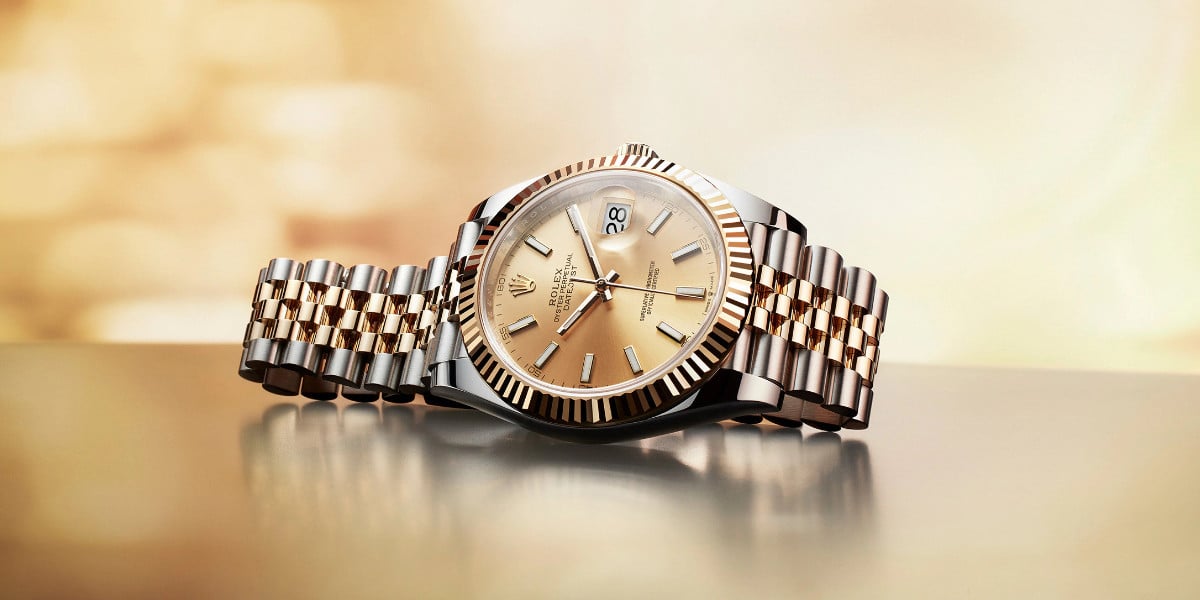This detailed photograph captures a sophisticated wristwatch, resembling a Rolex but likely a high-quality imitation. The watch boasts a beautiful seamless mix of gold and silver with a metal band. Prominently, the dial features a gold rim and a refined metal crown, along with the date marker displaying "28." The time on the watch shows approximately 1:50, indicated by the silver hands, with the second hand resting at the six o’clock position. The face of the watch includes a symbolic marker at the 12 o'clock position and markers instead of numbers for the hours, with more pronounced minutiae of "55," "50," and "60." The wristwatch rests horizontally on a glossy, reflective surface that appears to be gold-colored, creating a gleaming reflection underneath. The backdrop is softly blurred with a gold backlit effect, highlighting the elegance and luxurious appearance of the timepiece. Overall, the photograph encapsulates a visually appealing accessory displayed in a warm, golden ambiance.